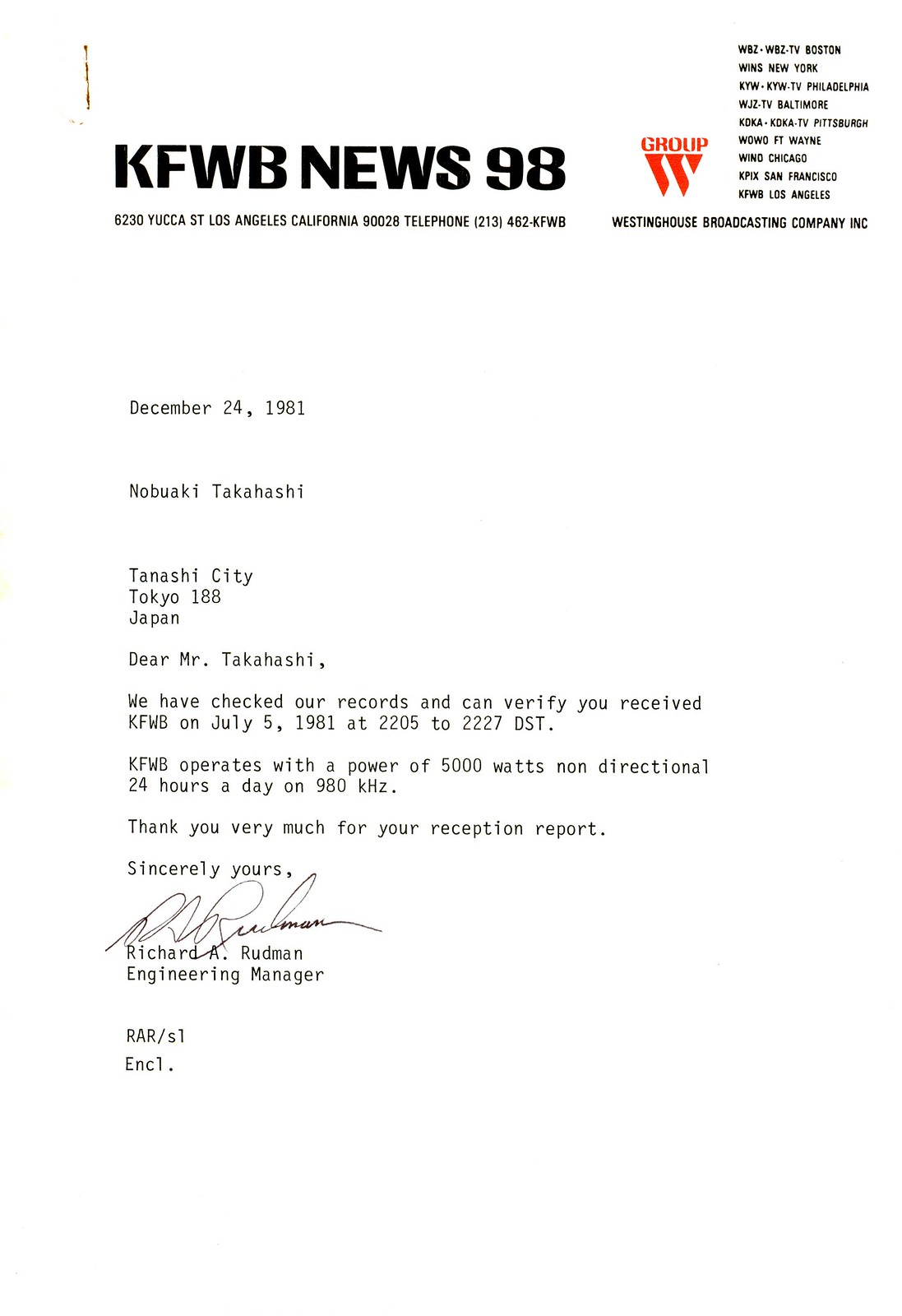This photograph captures a typed letter dated December 24, 1981, featuring the letterhead of KFWB News 98, located on Yucca Street, Los Angeles, California. The letterhead also includes the emblem of the Westinghouse Broadcasting Company, identified by a “W” symbol with the word "Group" above it. Addressed to Nobaki Takahashi in Tanashi City, Tokyo 188, Japan, the letter verifies that Mr. Takahashi received a broadcast from KFWB on July 5, 1981, between 2205 and 2227 DST. It details that KFWB operates with a power of 5,000 watts, non-directional, 24 hours a day on the frequency of 980 kHz. The correspondence is signed by Richard A. Rudman, Engineering Manager, with his name and title printed below his signature. The letter also includes an enclosure, denoted by the initials RAR-SL.